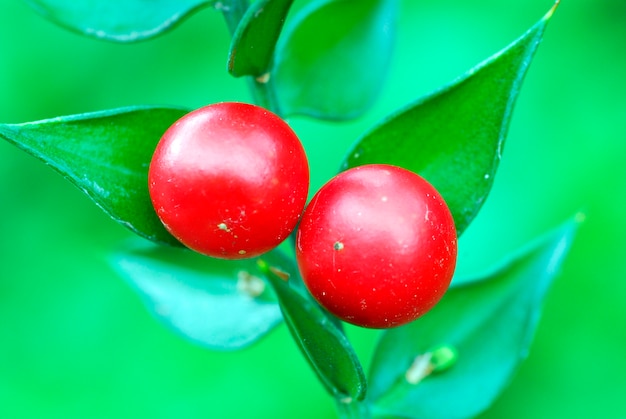This close-up photograph features two round, shiny, deep red berries, likely holly berries, nestled together on a stem amidst several distinctly pointed, emerald green leaves. The leaves, numbering about eight, are wide at the base and taper to sharp points. Some of these leaves have small droplets of water on them, adding to the fresh and vivid appearance of the image. The backdrop is a soft, out-of-focus, light green, which contrasts with the intense reds and greens of the berries and leaves, highlighting their vibrant colors.